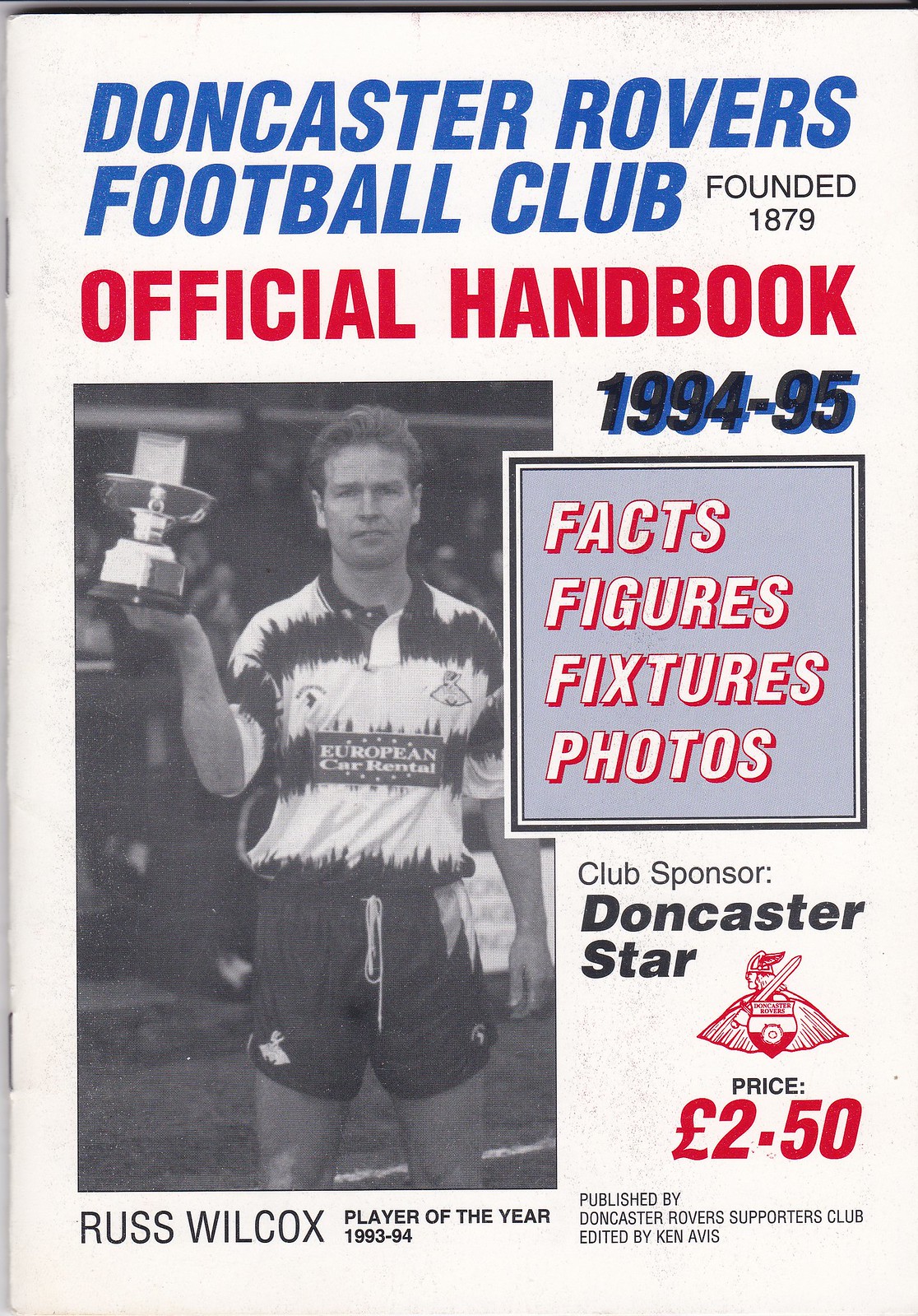The image is the cover of the "Doncaster Rovers Football Club Official Handbook 1994-95," published by the Doncaster Rovers Supporters Club and edited by Ken Avis. The cover has a white background with various colored texts. At the top, in blue font, it reads "Doncaster Rovers Football Club," followed by "Founded 1879" in black font. Below this, in red font, it states "Official Handbook," with "1994-95" in black font on a blue background.

On the left side of the cover, there is a black and white photograph of a soccer player identified as Ross Wilcox, the Player of the Year for 1993-94. He is white with short brown hair, and he is holding a trophy in his right hand. Wilcox is wearing a T-shirt that says "European Car Rental" and dark-colored short shorts. Under the photo, it states his name and title.

To the right of the photograph, within a blue square with a black border, white text outlined in red reads "Facts, Figures, Fixtures, Photos." Below this, in black font, it says "Club Sponsor Doncaster Star." The bottom of the cover indicates that the handbook's price is 250 pounds.